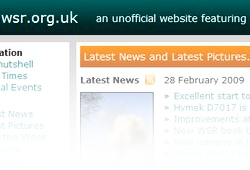The image captures the top section of a website. The header features a sleek black background that stretches horizontally across the top. On the left side of this black header, white text displays the URL "wsr.org.uk." On the right side, also in white text, the header states, "an unofficial website featuring."

Directly below the header, on the bottom left, part of a category section is visible against a white background. Adjacent to this section, there is a prominent orange rectangle with the words "Latest News" and "Latest Pictures" in bold white text. Beneath this orange rectangle, the phrase "Latest News, 28 February 2009" is displayed, followed by a series of light blue hyperlinks that appear to lead to different news articles.

As the image fades towards the bottom, the hyperlinks gradually disappear into a blank, white background, completing the overall composition of the image.